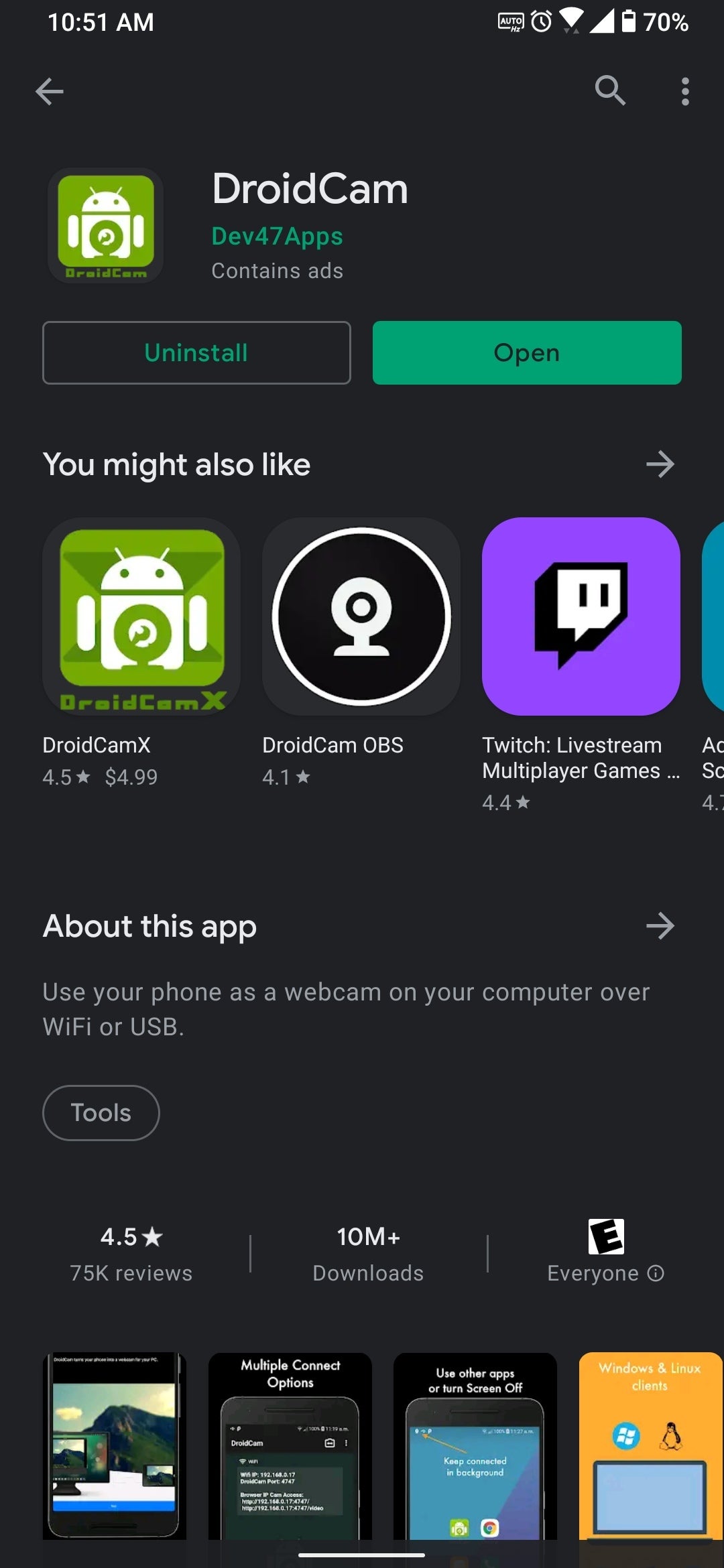The image showcases the DroidCam app as displayed on an app store platform. The screen has a black background with the time, 10:51 AM, displayed at the top left corner. To the right of the time are the connection icon and a battery icon indicating 70% charge. 

Just below, a left arrow icon appears on the left side, accompanied by a search bar icon and an icon with three vertical dots on the right side. The main content starts with the app name "DroidCam" accompanied by a logo depicting a white robot within a green square. Directly below the logo are buttons labeled "Uninstall" on the left and "Open" on the right, the latter highlighted with a green rectangular background.

Further down, under the section titled "You might also like," there are three suggested apps: DroidCam X, DroidCam OBS, and Twitch. Below these suggestions is a brief description categorized under "About this app," summarizing the app's functionality: "Use your phone as a webcam on your computer over Wi-Fi or USB."

The "Tools" section follows, highlighting the app's rating of 4.5 stars, its 10 million downloads, and its classification as suitable for everyone (E for Everyone). Finally, four images of app screens are displayed at the bottom: the first predominantly in white, black, and blue; the second black with white text; the third blue with white text at the top; and the last predominantly orange.